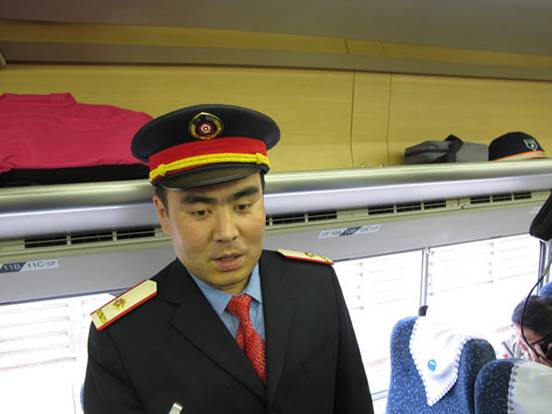A middle-aged Asian man, presumably in his 40s, dressed as a train conductor or bus driver, stands prominently in the left foreground of the image. He is wearing a black suit jacket adorned with yellow shoulder pads and is paired with a light blue collared shirt and a red tie. His black cap, detailed with a red and yellow band around the rim, sports a gold badge at the top. He maintains a neutral expression while looking slightly downward towards the camera. The background suggests the interior of a bus, characterized by a yellow wall, a mix of white and off-white sections, and a window running along the lower half. The bus seats, positioned in the bottom right corner, are blue with white coverings. Various items are visible, including a pink and black garment, a gray case with a black strap, and a dark hat with a white symbol and rim. The scene also features a silver vent below these items. An individual with dark hair talks on a black cell phone to the right, under a hanging black object. Overall, this bus interior is depicted with vivid details, potentially indicating its stationary state before departure.